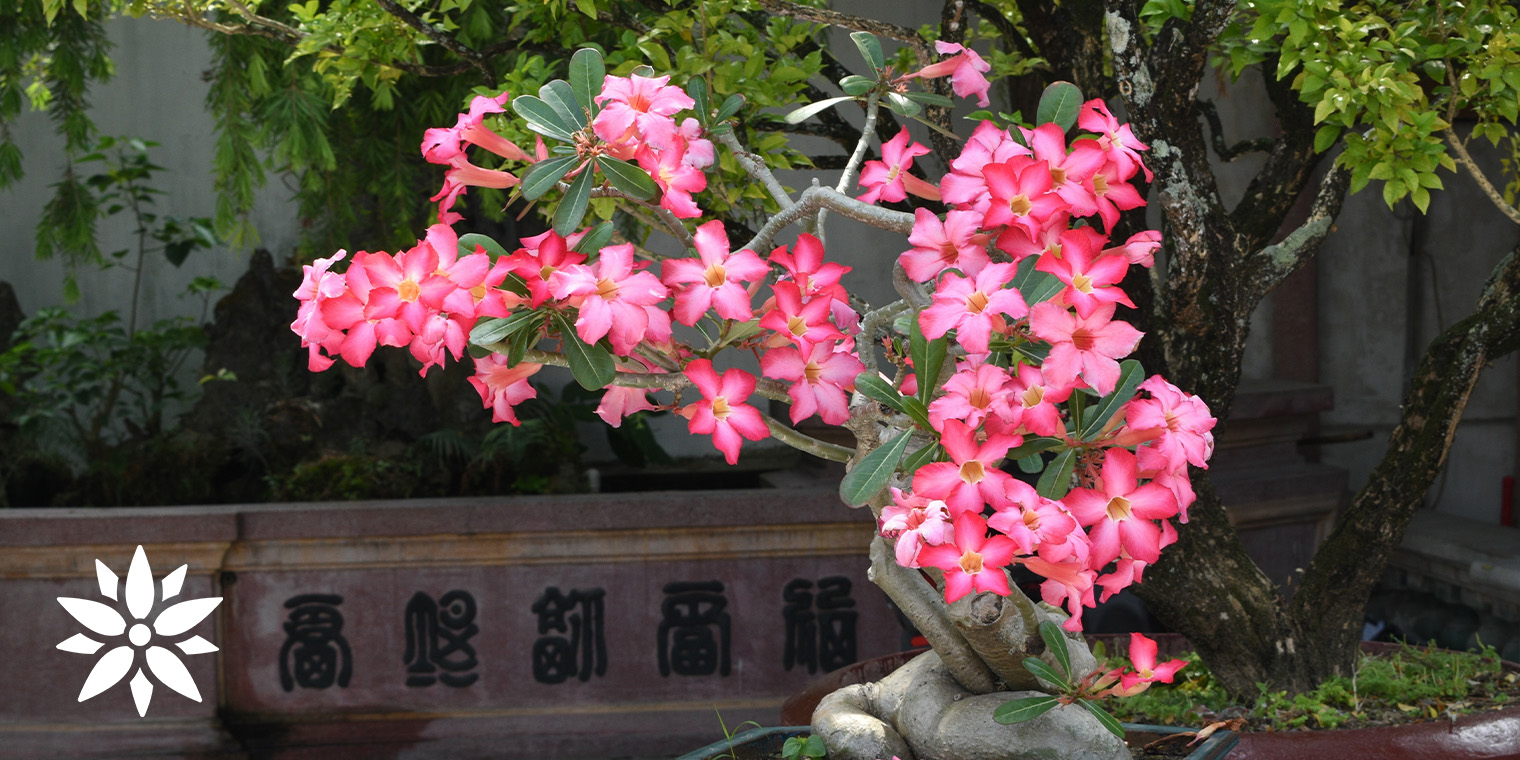The image showcases a vibrant garden dominated by a unique flowering plant that resembles a cactus due to its wide stem but is unlike any common species. The plant features an abundance of pink flowers, each with five petals that transition from a darker pink at the edges to a white center. The blossoms reveal intricate stamens at their core. The plant's substantial stem sprouts smaller leaves, which are elongated ovals, and these leaves extend from branches that originate from a wider section of the plant. The base of the plant displays gray, ooze-like roots, with the main stem angling up at a 45-degree slant from the ground. This central plant spans roughly the middle third of the image, stretching from one-third from the right edge to one-third from the left.

In the garden's backdrop, there is a gray stone wall adorned with five Japanese characters, adding an element of cultural detail to the scene. To the right of the primary plant is a secondary tree with a gray trunk, interspersed with patches of green moss and small leaves, extending up to the top of the image. The left bottom corner features a white flower logo with a star pattern nestled within another star outline, possibly indicative of a brand or garden logo. The entire scene is set against a well-lit backdrop, with additional foliage partially shaded and extending towards a distant stone wall. The text and design elements suggest an Asian, possibly South Asian, influence.